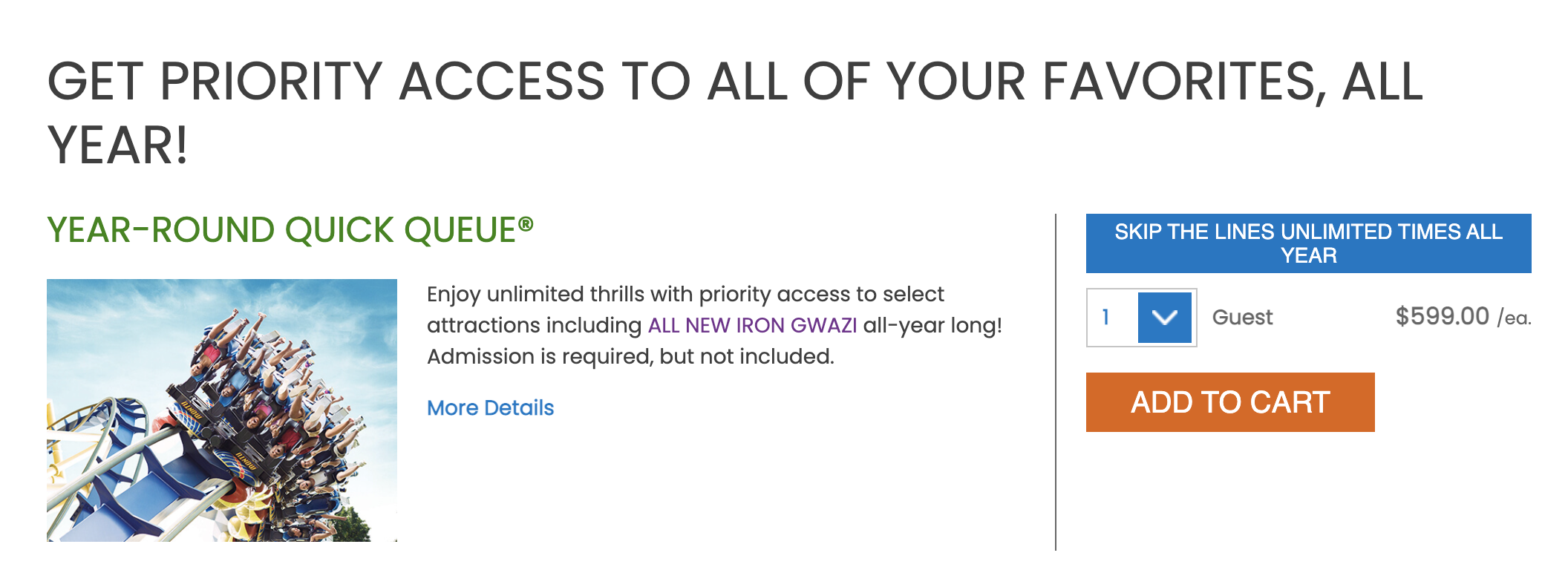The web page features a promotional offer at the top, proclaiming "Get Priority Access to All of Your Favorites, All Year." Highlighted in green text is the phrase "Year-Round Quick Queue." Dominating the visual space is a vibrant image of a roller coaster, colored blue and yellow, with riders depicted upside down, mouths agape in excitement, and legs dangling freely.

Accompanying this thrilling image is text detailing the offer: "Enjoy unlimited thrills with priority access to select attractions, including the all-new Iron Gwazi, all year long. Admission is required but not included.” Below this, a blue "More Details" button beckons further exploration. A black line separates this section from additional information indicating, "Skip the lines unlimited times all year."

A box allows users to adjust the number of guests with a white downward arrow next to the number 1. The price is listed as $599 per person for the entire year. An orange "Add to Cart" button facilitates the purchase. The overall design maintains a clean aesthetic with a white background and black text, punctuated by various interactive buttons, and of course, the dynamic roller coaster image.